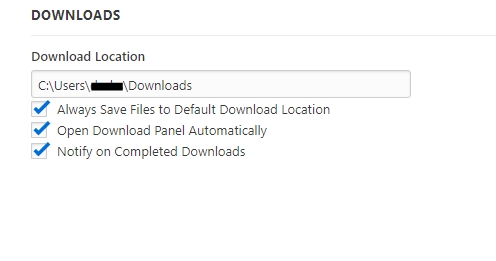The image is a horizontally rectangular screenshot with a plain white background, depicting a section of a downloads settings interface. In the upper left corner, bold capital black letters spell out "Downloads." Directly below, a thin horizontal gray line serves as a divider. Further down, the label "Download Location" is displayed, followed by a text field containing the path "C:/Users/[blacked out]/Downloads." Below this text field, there is a vertical list of three settings options, each accompanied by a checkbox on the left side. All three checkboxes are ticked. The listed options from top to bottom are: "Always save files to default download location," "Open download panel automatically," and "Notify on completed downloads."